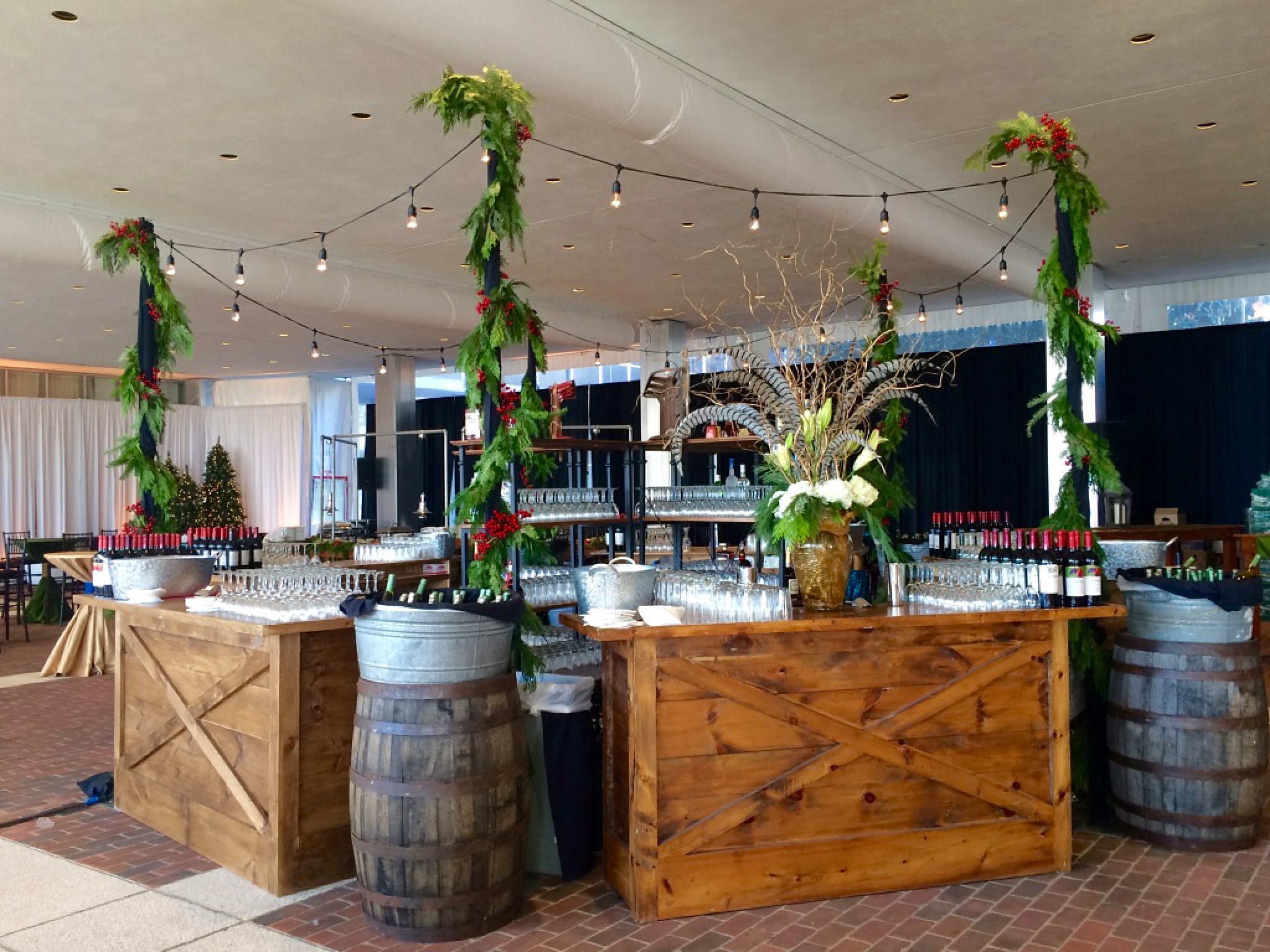The photograph captures a cozy, makeshift bar setup inside a room, evoking a warm and festive atmosphere. The bar is assembled with rough wooden tables, featuring sturdy wooden boards arranged in an X-pattern. Dark wooden barrels, contrasting with the lighter wood of the countertops, are scattered around, some topped with wine bottles and glasses. The ceiling, an off-white color, adds to the rustic charm, while brick and dark gray tiles cover the ground below. Poles adorned with wreaths of red flowers or berries rise up from the tables, draped with delicate string lights giving off a bright white or soft yellow glow, reminiscent of outdoor settings. To the right, a black wall provides a striking backdrop, partially covered by white curtains towards the center-left. A touch of holiday spirit is evident with a beautiful flower centerpiece and Christmas decorations, including a Christmas tree in the back, creating a thoroughly inviting and celebratory scene.